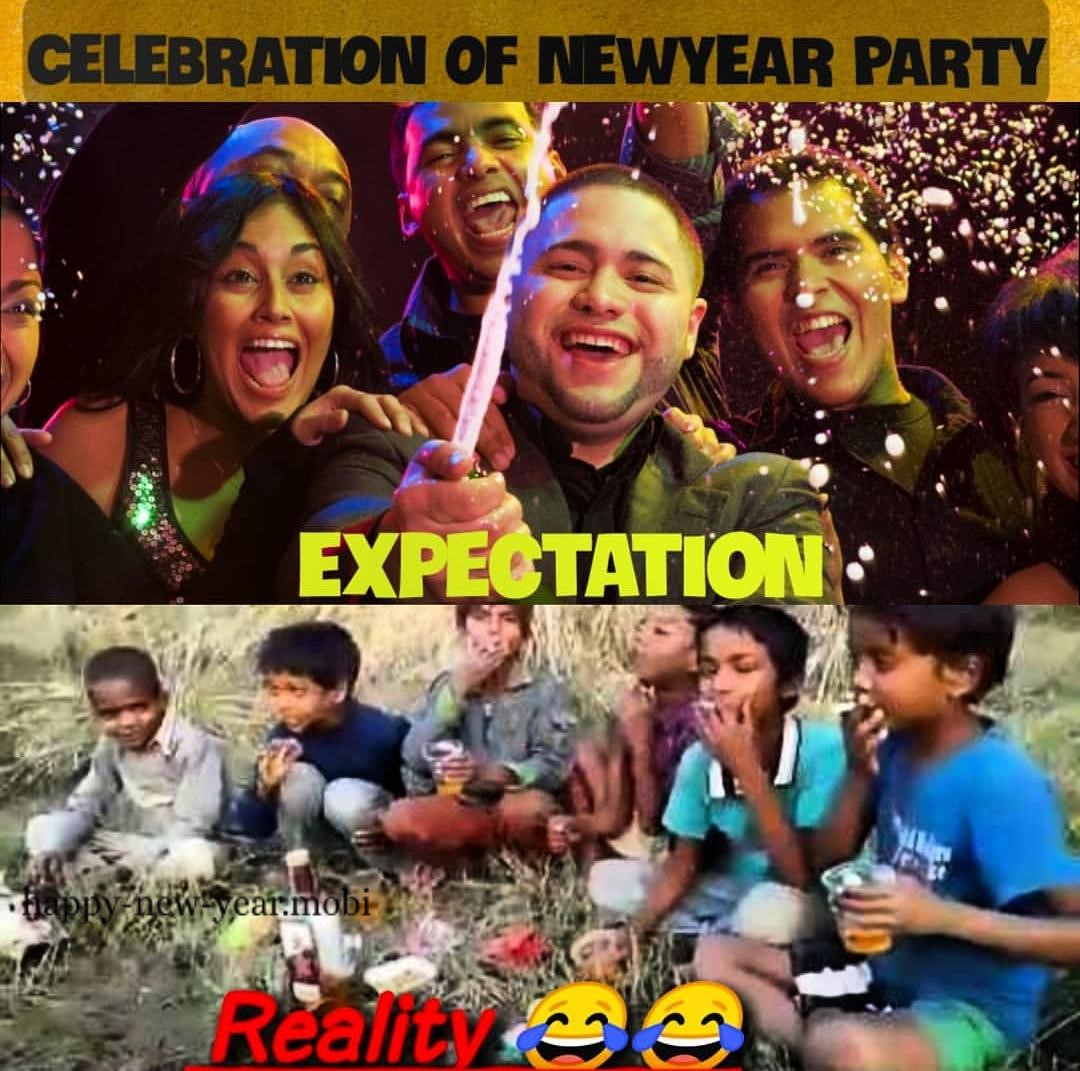The image consists of two panels, each conveying a contrasting depiction of New Year's celebrations. The top panel, set against a dark gold-colored background, features bold black letters reading "Celebration of New Year Party". Below this text, a lively scene unfolds with several adults laughing, holding party favors, and surrounded by champagne and alcohol droplets spraying through the air. This image captures an atmosphere of joy and exuberance, with people smiling, cheering, and their mouths open in delight. At the bottom of this panel, the word "Expectation" is highlighted in bright yellow capital letters.

The bottom panel, of equal size to the top one, offers a starkly different scene labeled "Reality" in bold red letters, accompanied by two laughing emojis with tears. This image shows six boys sitting in a field of rusty grass, holding cups that might be mistaken for cigarettes from a distance. Their attire includes a mix of blue t-shirts and collared shirts. The boys appear more subdued, focused on eating snacks during what appears to be a casual picnic. On the left side of this panel, there is text reading "happy-new-year.MOBI," adding a digital touch to the contrasting imagery. 

Together, the two panels create a humorous juxtaposition between the high-spirited expectations of a New Year's party and the more mundane reality of a simple outdoor meal.